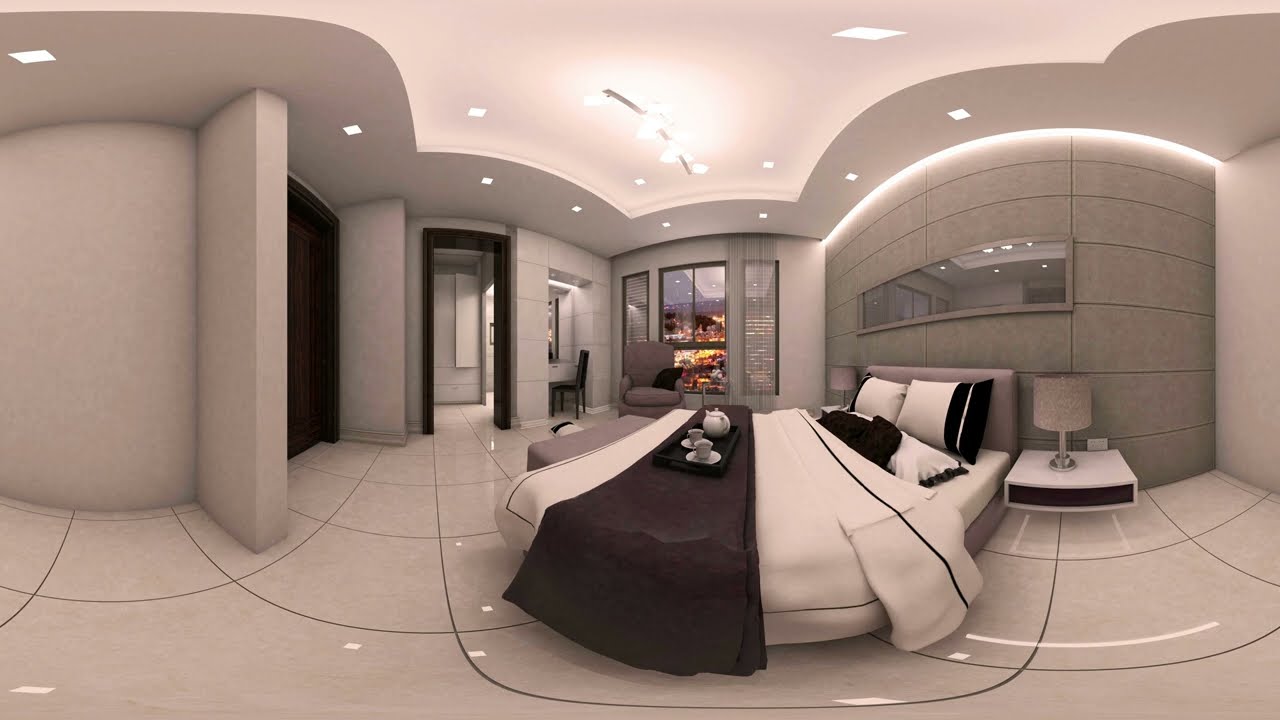The image is a fisheye-lens photograph of a luxurious and modern bedroom, possibly in a high-end apartment or penthouse. The bed, meticulously made with black and white pillows and a white blanket, features a gray blanket stretched across it and a tray set with a white china teapot and two white cups and saucers. There's a lamp on a black and white nightstand adjacent to the bed. The sleek white tile flooring, reflecting the recessed ceiling lighting, and the concrete walls give the room a contemporary feel. The room includes a curved wall and a shelf with a short lamp to the right. Floor-to-ceiling windows in the background offer a view into the city, adding a splash of color to the primarily monochromatic interior. The presence of multiple windows and doorways further emphasizes the room’s spacious and upscale ambiance.